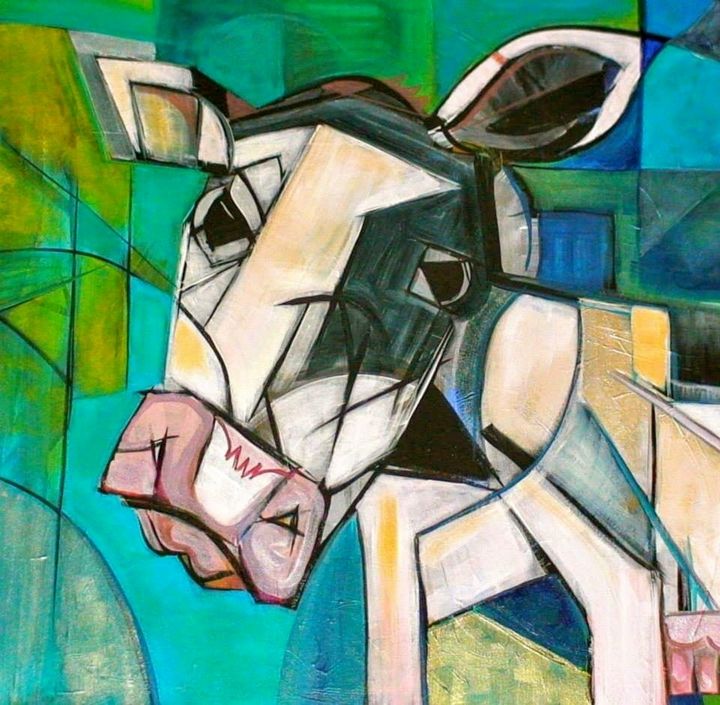The image depicts an abstract, Picasso-esque painting of a black and white cow, composed predominantly of geometric shapes. The cow stands out against a vibrant background of turquoise and yellowish-green hues, which gives the impression of stained glass or an abstract representation of an open sky with trees. The cow's head, tilted slightly to the left, directly engages the viewer with its triangular, black eyes. Its snout, a pink-reddish color, is prominently featured along with its erect, attentive ears. The cow's face is mostly white with a distinctive black patch around its right eye and a white stripe between its large pink nostrils. The body of the cow, visible in parts, shows a mix of black and white with sections of yellow and blue above the chest and an additional blue patch near its shoulder. The entire composition emphasizes the abstract and conceptual nature of the cow, using a variety of lines, curves, and diagonal shapes to create a striking and unique piece, devoid of any artist's signature.